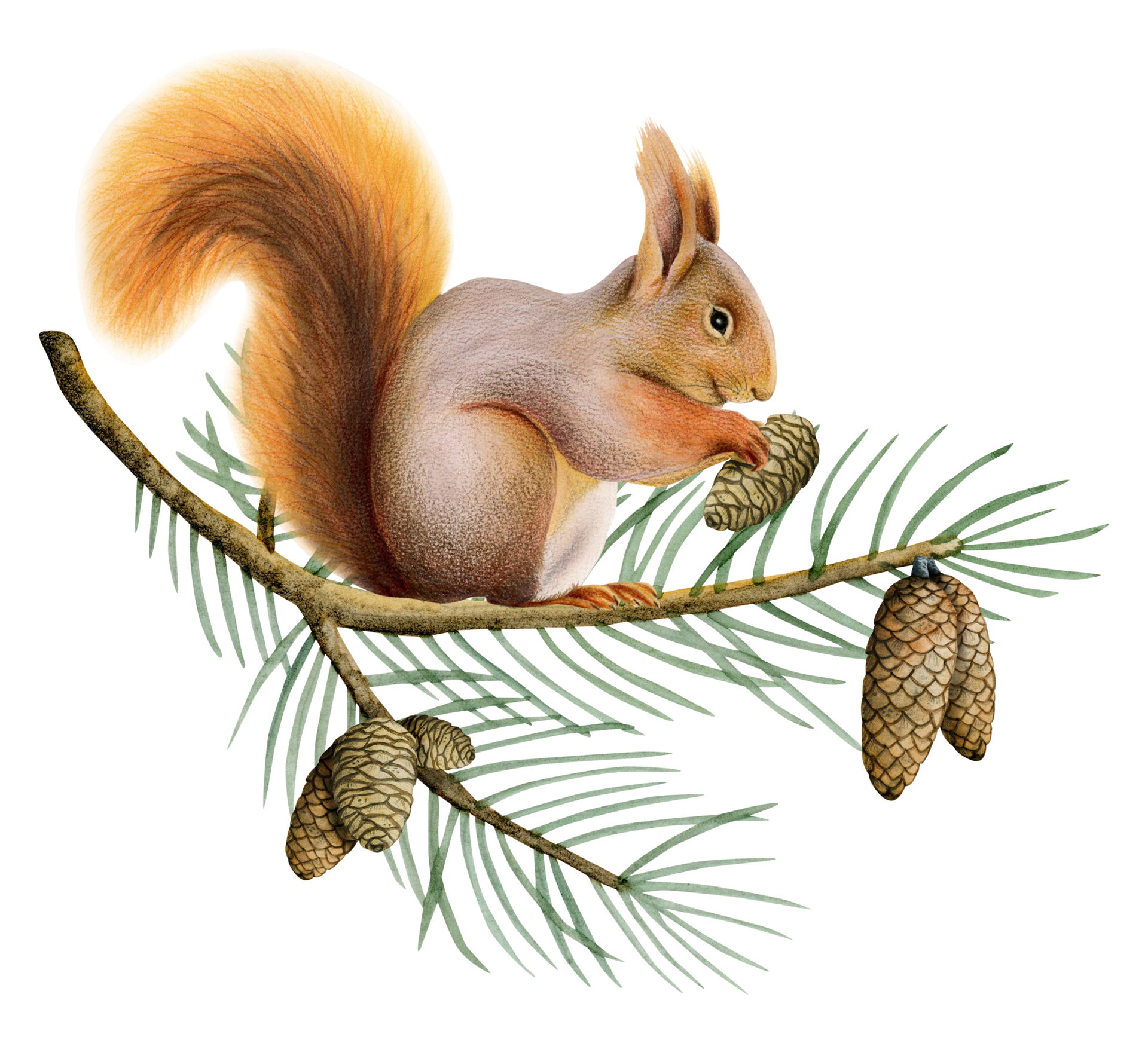The illustration depicts a happy, vintage-style squirrel with pointed, upright ears and a fluffy, curving tail that is a mix of orange and brown hues. The squirrel's body boasts a blend of gray, yellow, and orange tones, tapering to white on its stomach area. This detailed colored pencil drawing features the squirrel perched on a slightly upward-curving pine or conifer branch, meticulously shaded with tones of pale sap green and beige-tan pine cones. The squirrel is captured in a moment of poised anticipation, holding a small pine cone in its right paw and gazing down at it with its black eyes, which have tiny white highlights. Surrounding the squirrel and accentuating the scene are multiple pine cones; two larger ones dangle at the front of the main branch, while a cluster of three hangs from a lower bough. The squirrel is centrally positioned against a stark white background, highlighting the intricate textures and shading of its fur and the branch it inhabits. This charming and whimsical scene exudes a classic, nostalgic charm.